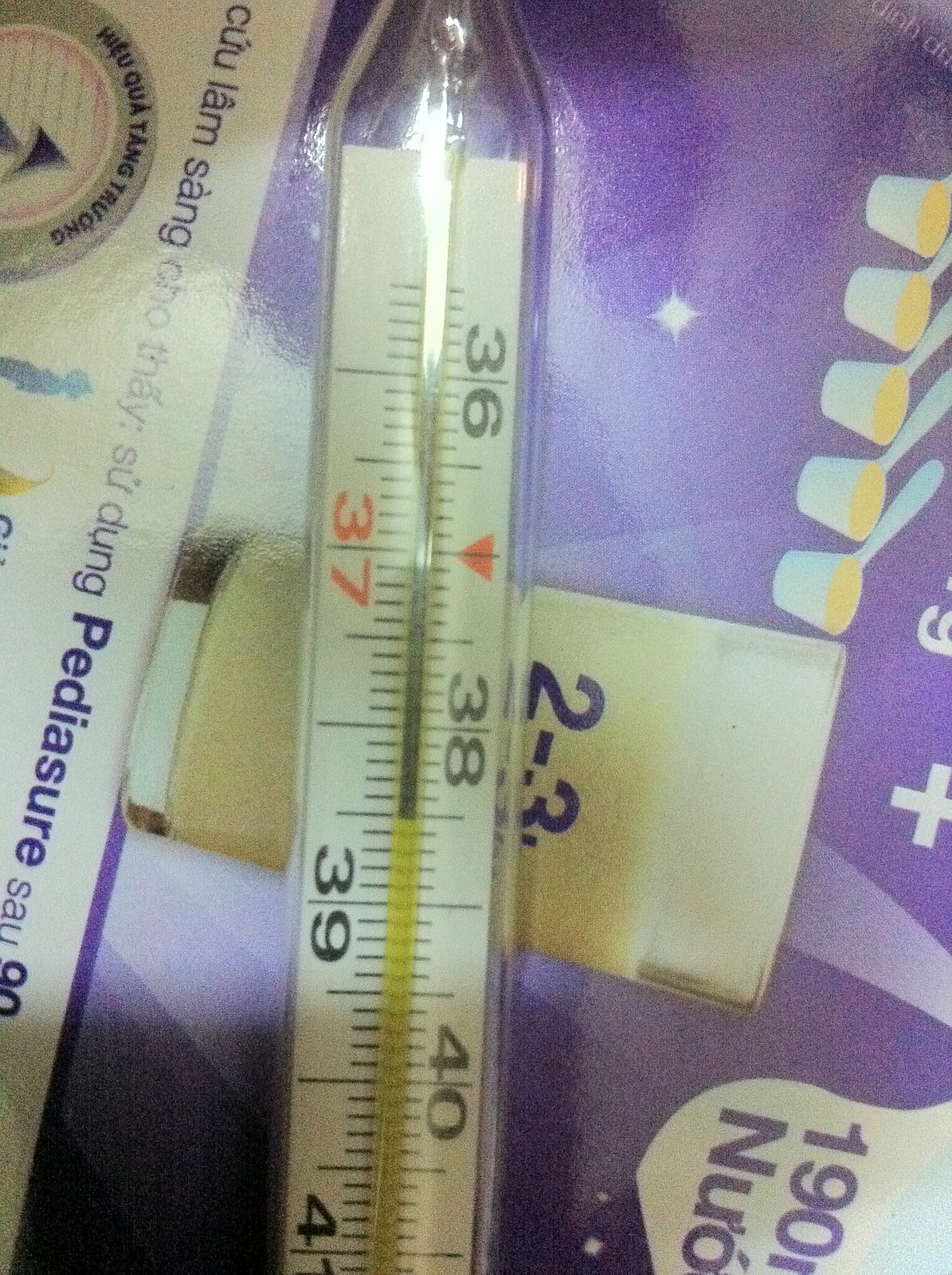The image features a translucent glass thermometer prominently displayed in the center. The thermometer has readings marked from 36 to 41, predominantly in black, except for the number 37 which is highlighted in red with a red arrow pointing downwards above it. The center of the thermometer houses a meter colored in yellow and silver. The thermometer rests on a piece of paper that is purple and white, adorned with text in a foreign language.

In the background, there is a cup with the numbers "2" and "3" displayed together, and it contains a cream-colored liquid. A subtle, almost square-shaped shadow appears in the bottom left corner of the image. In the bottom right corner, the number "190" is visible. Toward the top right, five spoon-shaped objects filled with a yellow liquid and colored light blue are arranged neatly.